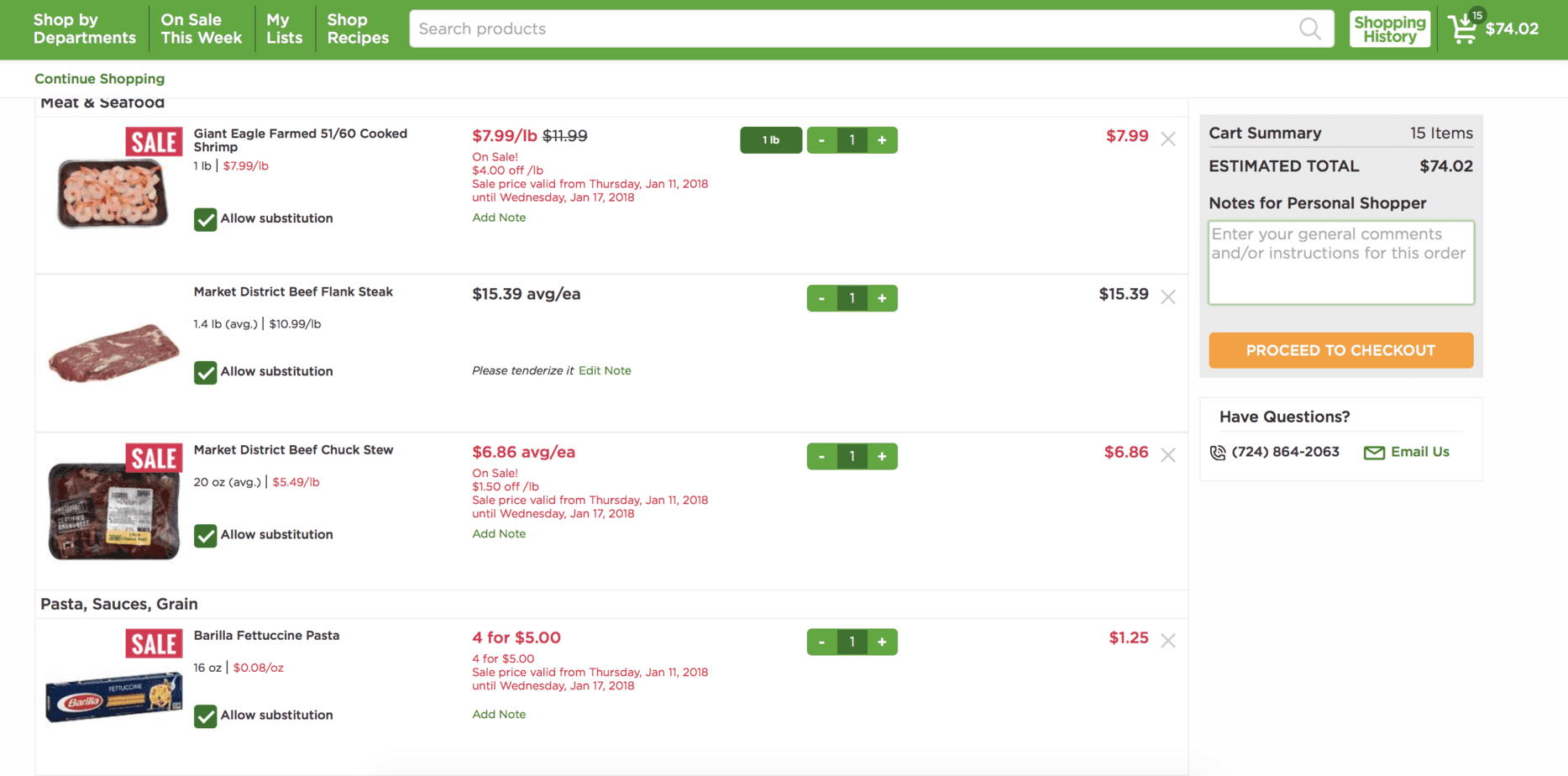The image is a detailed screenshot of an online grocery shopping webpage. At the top of the page, a prominent green banner features white text along with several tabs for navigation. These tabs include "Shop by Departments," "On Sale This Week," "My Lists," and "Shop Recipes." Beneath the banner, a rectangular search bar with the placeholder text "Search products" is accompanied by a magnifying glass icon.

A white box with green text labeled "Shopping History" is situated below the search bar. Nearby, a cart icon indicates that 15 items are in the cart, with the estimated total amounting to $74.02. This information is reiterated in a grey box labeled "Cart Summary," which also includes space for "Notes for Personal Shopper," where users can enter their general comments or instructions for the order. An orange button labeled "Proceed to Checkout" is prominently displayed.

The cart contains several selected items, including Giant Eagle Farmed Cooked Shrimp priced at $7.99 per pound, Market District Beef Flank Steak for $15.39, Market District Beef Chuck Stew at $16.86, and Barilla Fettuccine Pasta available in a deal of $4 for $5.